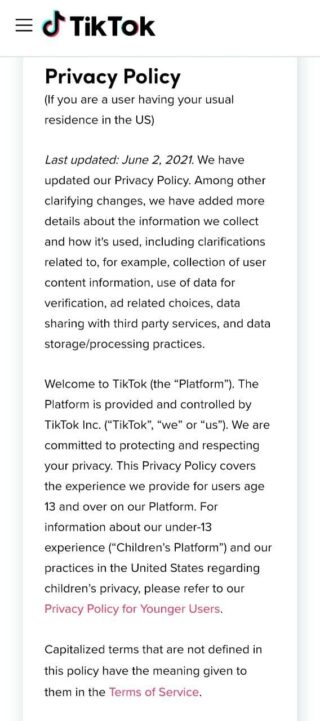The webpage shows a privacy policy for TikTok, prominently displayed with a bold black header that reads "TikTok" accompanied by three horizontal lines on the left. Below the header, it states "Privacy Policy" with a note clarifying it applies to users residing in the U.S. The policy's last update is marked as June 2nd, 2021.

The introductory text informs users about recent updates to the privacy policy, highlighting that more details have been added regarding the information TikTok collects and uses. This includes specifics on the collection of user content information, data use for verification purposes, choices related to advertisements, sharing of data with third-party services, and practices regarding data storage and processing.

The page welcomes users to TikTok (referred to as 'the platform'), which is managed by TikTok Inc., emphasizing their commitment to respecting user privacy. The policy specifically covers users aged 13 and over. For users under 13, there is a separate privacy policy, highlighted in red, which addresses practices related to children's privacy in the United States.